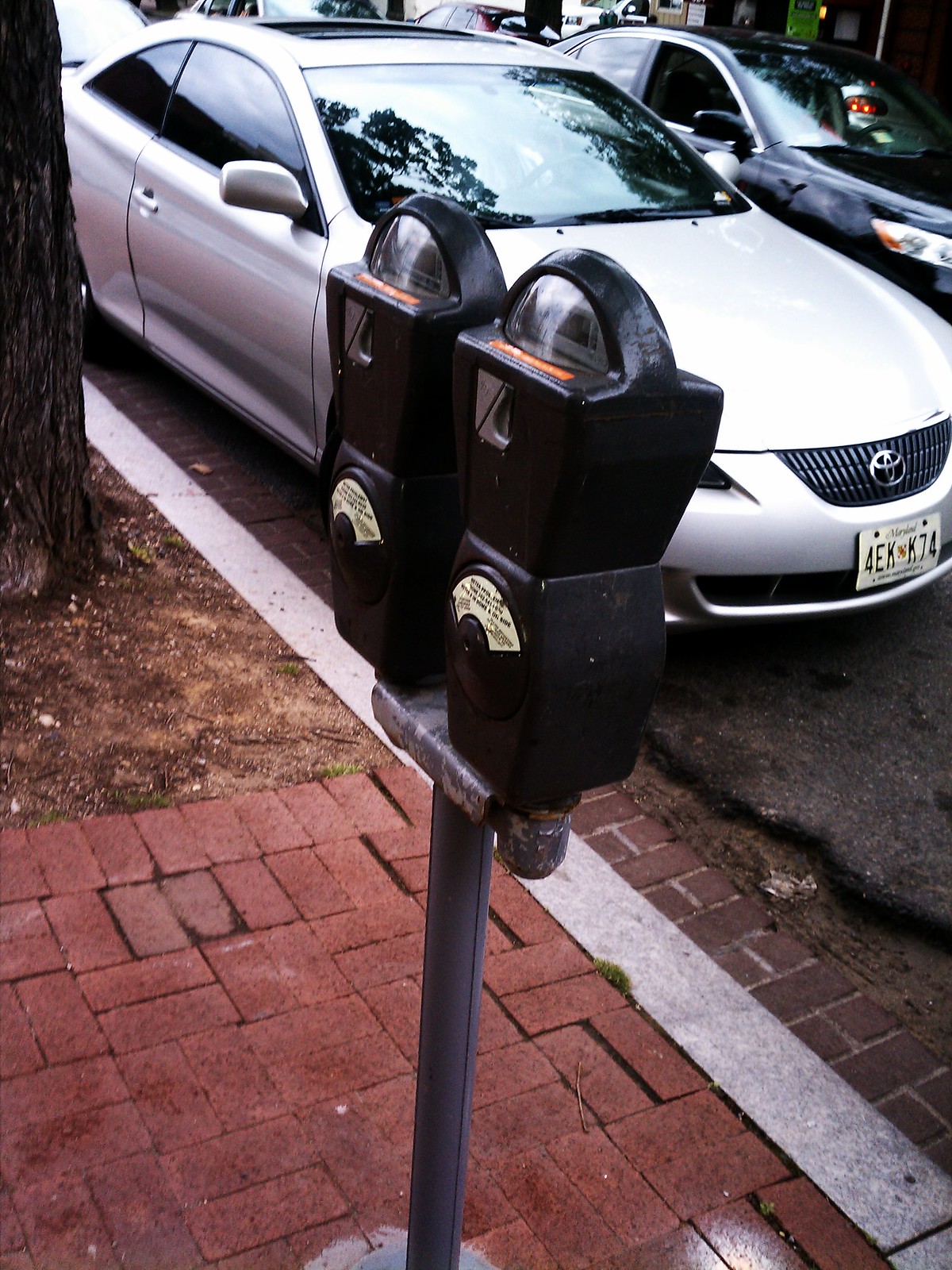This image captures a city street scene with various details that draw the viewer's eye. In the forefront, there's a dual black parking meter mounted on a gray pole, situated on a red brick walkway that extends past the curb, transitioning into a broken, rough-looking asphalt street. Parked closest to the meter is a white car, likely a Saturn or Toyota, with license plate number 4EKK74, which appears to be from Maryland. Adjacent to the white car is a black vehicle with its window open. Additional cars can be seen both parked along the street and driving in the background. To the left of the frame, there's a tree with dark brown and grayish bark, surrounded by a mix of dark and light brown dirt.